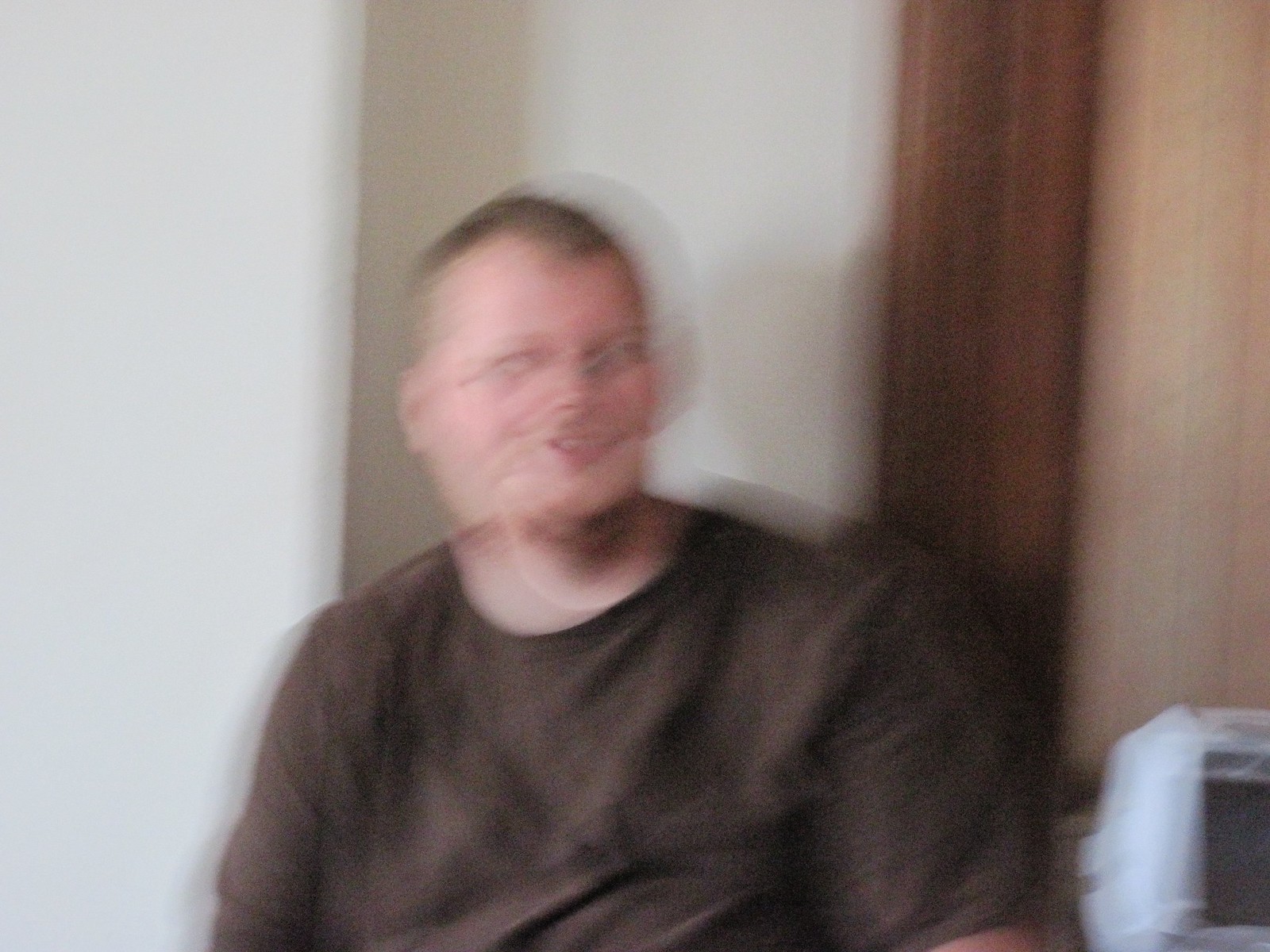A blurred image captures a broad-shouldered, large man who seems to be smiling, despite the indistinct quality of the photo obscuring his facial features, including his eyes. He is seated, wearing a loose-fitting dark shirt that appears to be either black or dark brown. To his side, there's an item with a white frame; its exact nature is ambiguous as it could be a computer, a can opener, or a picture frame. The setting features an off-white wall with a wooden section leading to a beige-toned wallpaper in the background.